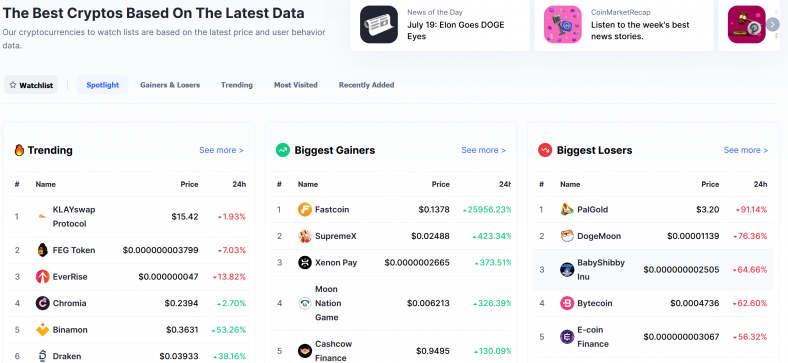The web page showcases various cryptocurrencies and their performance metrics, categorized to help users make informed decisions. Titled "The Best Cryptos Based on the Latest Data" at the top left, it provides easy navigation with two linked options: "News of the Day" and "Coin Market Recap." Users can explore multiple sections such as Watchlist, Spotlight, Gainers and Losers, Trending, Most Visited, and Recently Added. Currently, the Spotlight page is highlighted.

The page is divided into three main columns, each representing a distinct category. The "Trending" section displays six cryptocurrencies, with an equal split of three in red (indicating loss) and three in green (indicating gain). Adjacent to this, the "Biggest Gainers" section lists five cryptocurrencies, all marked in green to signify their upward movement. On the far right, the "Biggest Losers" section also contains five cryptocurrencies, all shown in red, reflecting their downward trend. Each section is uniformly sized, providing a clear, concise overview of the top-performing and underperforming cryptocurrencies.